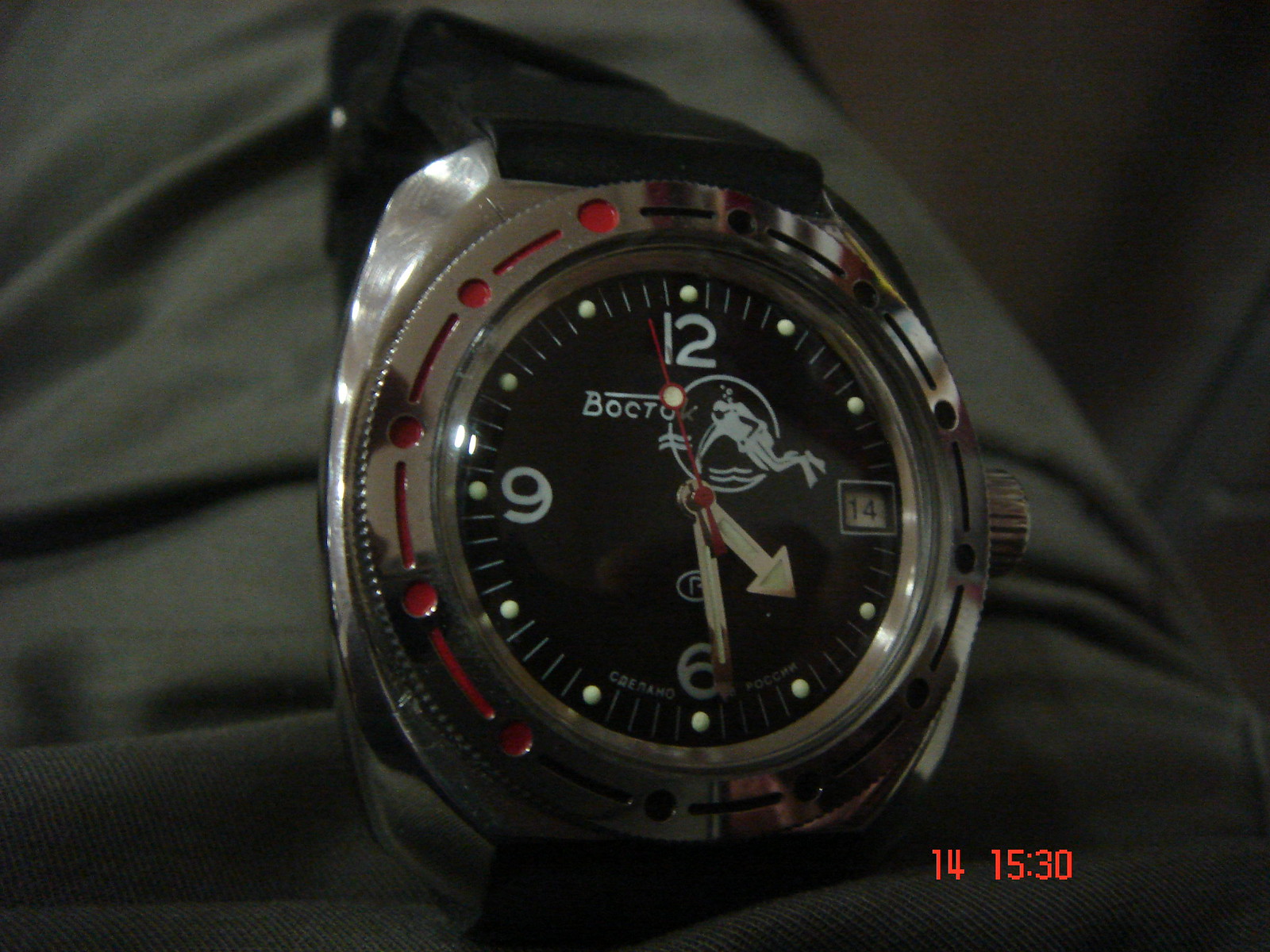This photograph presents a detailed, angled close-up of a wristwatch resting on a gray pair of pants. The watch features a sleek black band and a robust silver casing. The face of the watch is marked with a striking design, including a silver outer ring. Notably, the left side of the watch face is accented with red dots and lines, while the right side is embellished with black. The watch includes a black face with luminous white dots around the perimeter for easy visibility in the dark, alongside the numbers 12, 6, and 9 in white. At the 3 o'clock position, a small white square displays the date as '14' in black. The hands of the watch are silver, with glow-in-the-dark lines, and the second hand is red, featuring a glowing white dot near its tip. The brand name 'Bachtok' is inscribed on the watch face, and there is an image of a diver encircled by water, suggesting water resistance. Additionally, a digital stamp in the bottom right corner of the image shows the date '14' and the time '1530' in red font.